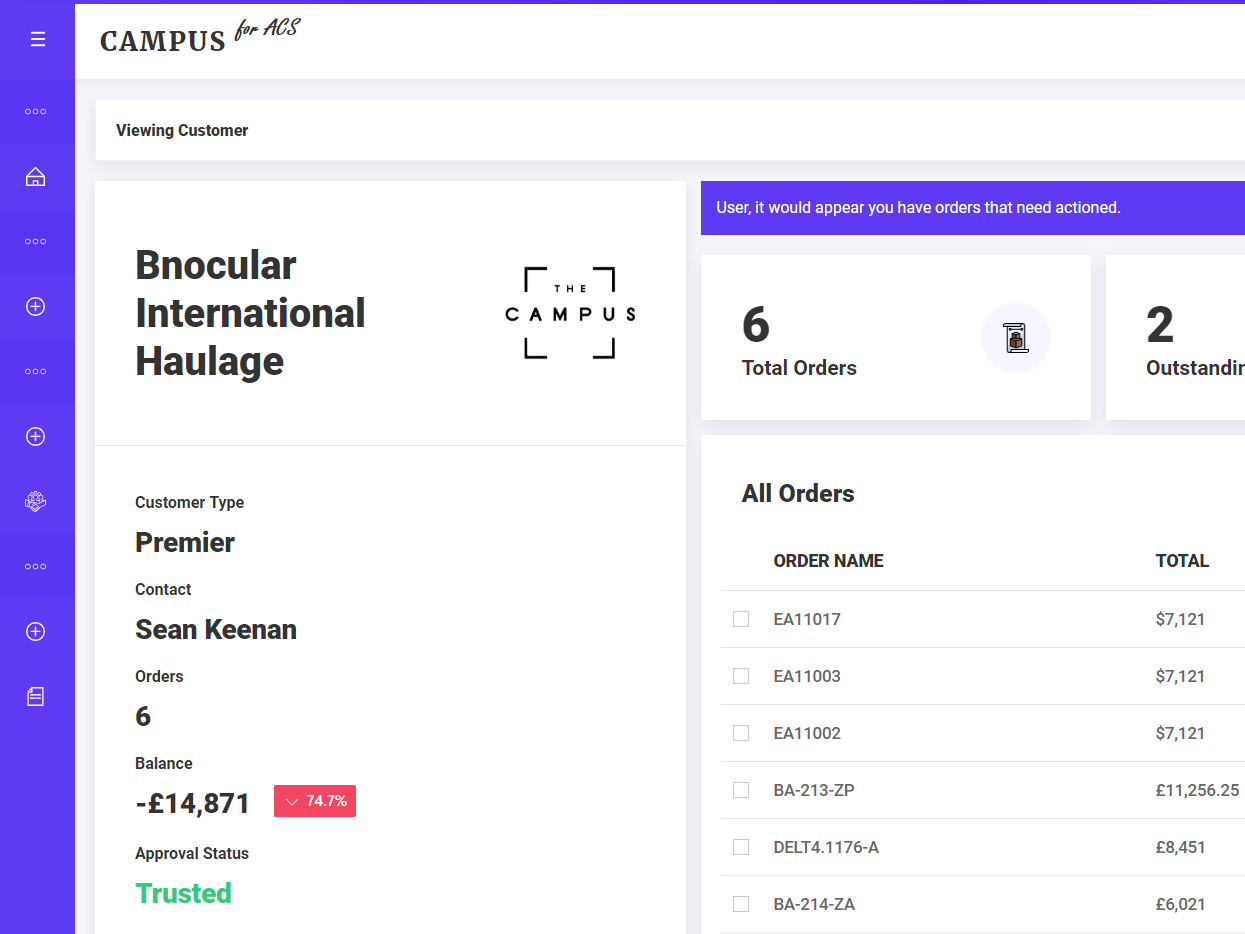The screenshot showcases a user interface designed for managing customer orders. The left side of the screen features a vertical blue toolbar with various icons arranged in a linear sequence. From the top, these icons include three horizontal lines (menu), an indiscernible symbol, a home icon, another indeterminate symbol, followed by three plus symbols interspersed with another unrecognized icon, and finally, a document symbol.

Prominently displayed near the top center of the screen, the header reads "Viewing Customer." Below this, housed in a blue box with white text, a notification states, "User, it would appear you have orders that need action."

The interface then displays information pertaining to "Binocular International Haulage." Adjacent to this, a labeled box reads "The Campus." To its right, another box summarizes order statistics: "Six total orders," with "Two outstanding." Further down, additional details are provided in another box under "Binocular International Haulage," specifying customer type as "Premier," contact person "Sean Keenan," total of "six orders," and a negative balance of "£14,871."

A pink box with a downward-pointing arrow indicates a "74.7% approval status," while nearby, a green label confirms the customer as "Trusted."

Below these sections, a table lists order details under the headers "All Orders," "Order Name," and "Total." Each order is detailed with a unique code (e.g., "EA 11017") and corresponding total amount (e.g., "$7,121"). Accompanying each order code are checkboxes for selection.

The overall background of the interface is white, and the design elements suggest a clean, organized layout aimed at providing clarity and efficient navigation for the user.